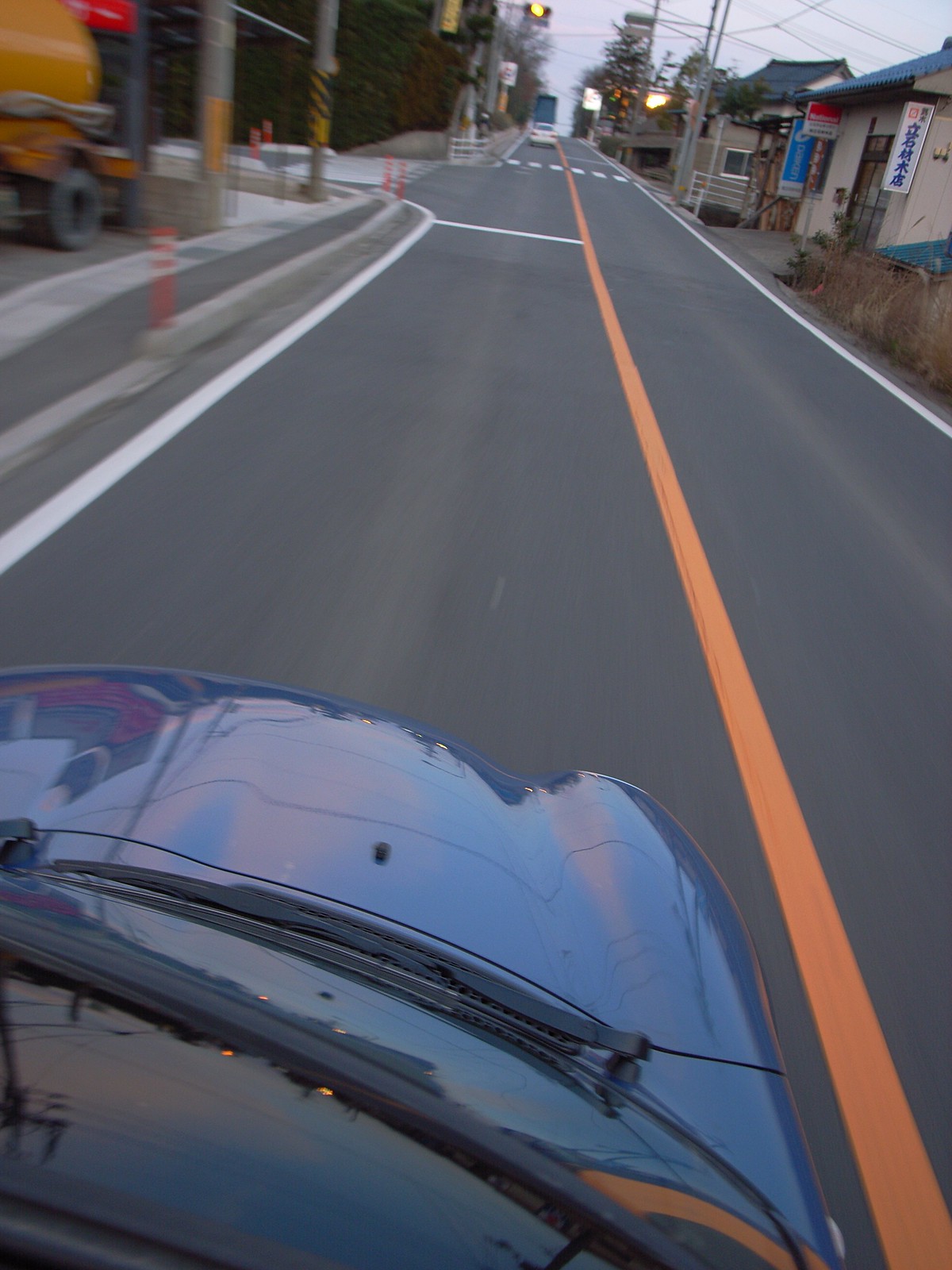An overhead photograph showcases a vibrant blue compact car driving down a narrow two-lane road. The image, likely captured by a drone or a high-reaching selfie stick, offers a unique top-down perspective. The car is positioned in the left lane, revealing the top of its windshield and a windshield wiper on the right side. The road is marked by a solid yellow stripe down the center and white stripes along its edges. On the right side, rows of houses are visible, while the left side features the rear end of a large yellow tanker truck. Two orange traffic cones are situated at a corner in the background, near two metal poles. In the distance, another building can be seen on the left side of the road. A traffic light hangs at the top center of the image, displaying a yellow signal, adding to the detailed urban scene.